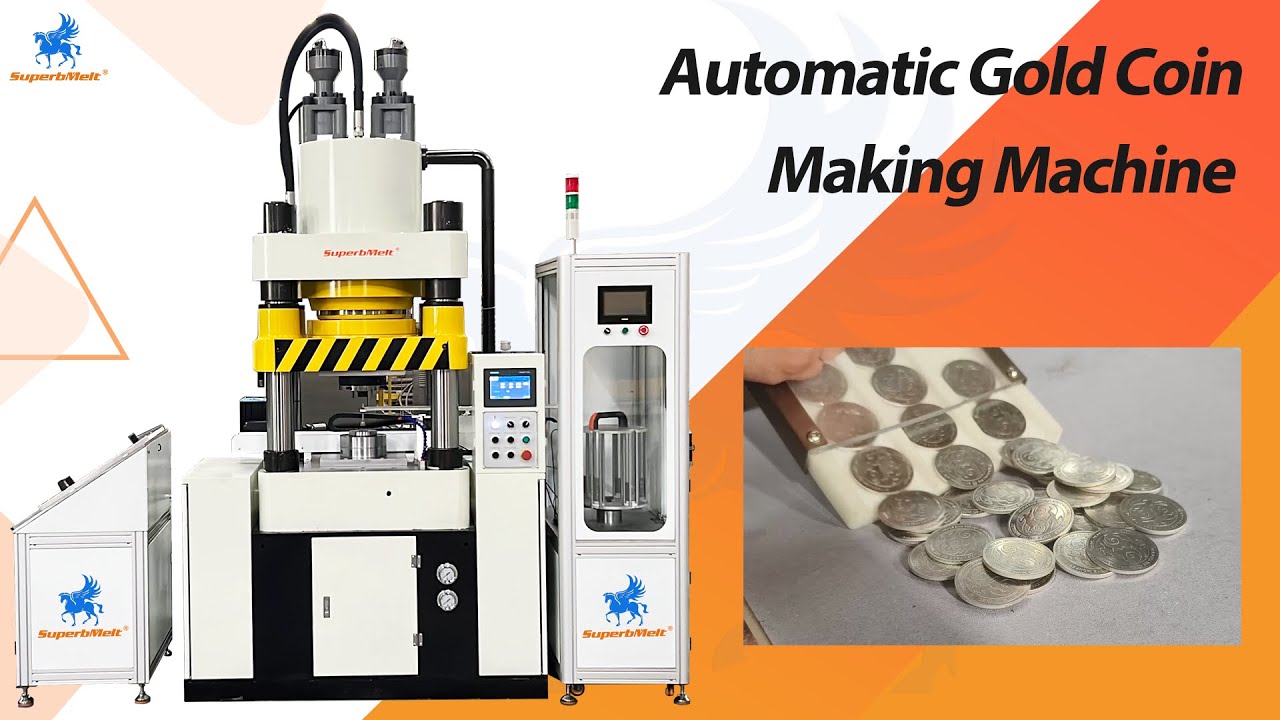The image features a detailed, multi-shaded background incorporating colors such as white, light pink, orange, and yellow. Dominating the left side is a substantial machine with three main components: a central unit flanked by smaller sections on both sides. The machine, primarily white with metallic highlights, includes various parts like pipes, rotators, buttons, a display screen, dispensers, and small cabinets, suggesting sophisticated mechanics, possibly involving hydraulic presses. Notably, it features yellow and black accents.

This equipment, identified as a coin-making machine, is branded as "Superb Melt" (stylized as S-U-B-E-R-B-M-E-L-T in red letters), accompanied by a blue Pegasus, or winged horse, logo that appears both on the machine and in the top left corner of the image. The right side of the poster prominently displays the text "automatic gold coin making machine" in black letters. Additionally, an inset image at the bottom right shows a glass-encased pouch from which gold coins are being poured onto a grey surface. Despite some silver coins depicted, the machine's primary advertised function is to produce gold coins.